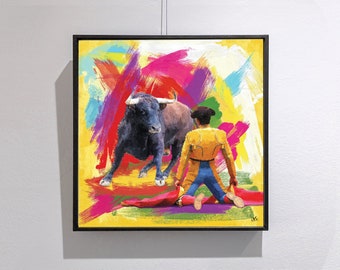A square painting, framed in black, is hanging on a white wall. The painting, created with vibrant and heavy brushstrokes, showcases a dramatic scene filled with color and motion. At the center of the composition, a matador on his knees, dressed in a gold or yellow jacket and blue pants with gold stripes, is holding a red flag or blanket in both hands. The matador, whose face is not visible, wears a traditional brown matador's hat. In front of him, a large brown and black bull with prominent horns is poised, seemingly ready to charge. The background is adorned with bold and expressive brushstrokes in a spectrum of colors, including fuchsia, purple, yellow, blue, green, orange, pink, red, and white, which amplify the sense of tension and movement in this powerful depiction.